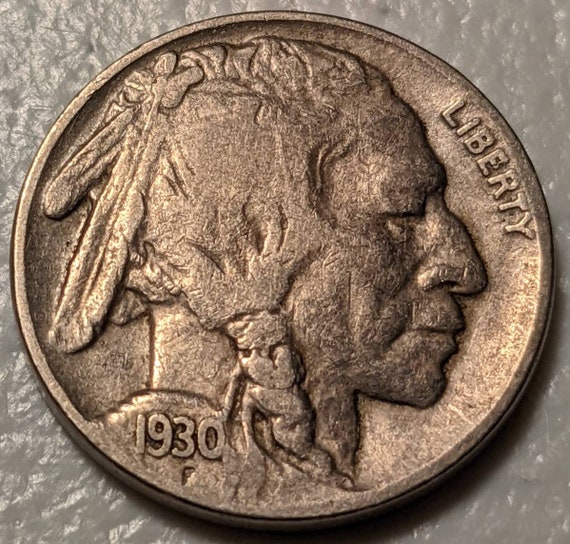This image features a worn 1930 Indian Head nickel, also known as a Native American head nickel, prominently centered against a semi-transparent, bumpy, gray background. The coin, silver in color but tarnished with age, appears dull and rusted. The design shows a right-facing Native American profile with faded hair details. At the top right edge, in sloping, all-capital letters, is the word "LIBERTY". The date "1930" is stamped at the bottom left of the coin. The image captures the coin's circular, slightly indented surface with a raised design, photographed from a top-down perspective, with equal spacing around the borders, suggesting careful framing in an indoor setting.